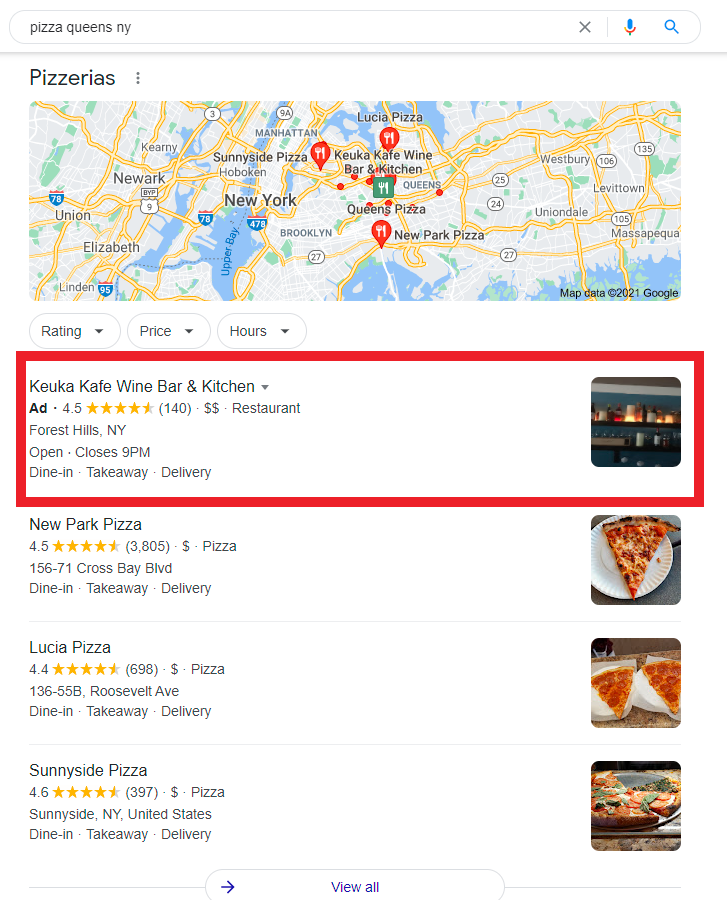Screenshot of Google search results for "Pizza Queens NY."

At the top of the screenshot, the Google search bar displays the query "Pizza Queens NY." Directly below the search bar is a grey divider line. Underneath the divider, the heading "Pizzerias" is visible with a vertical three-dot menu option beside it.

Following this, there is a map indicating New York City with three red pins marking specific pizza places. Under the map, there are three drop-down buttons labeled "Rating," "Price," and "Hours" for filtering the search results.

Highlighted in a thick red border, an advertisement for "KUKA Cafe, Wine and Bar, and Kitchen" captures attention. Below the ad, the search results include listings for "New Park Pizza," "Lucia Pizza," and "Sunnyside Pizza." Each listing features the pizzeria's name, star rating, address, and icons indicating dine-in, takeaway, and delivery options.